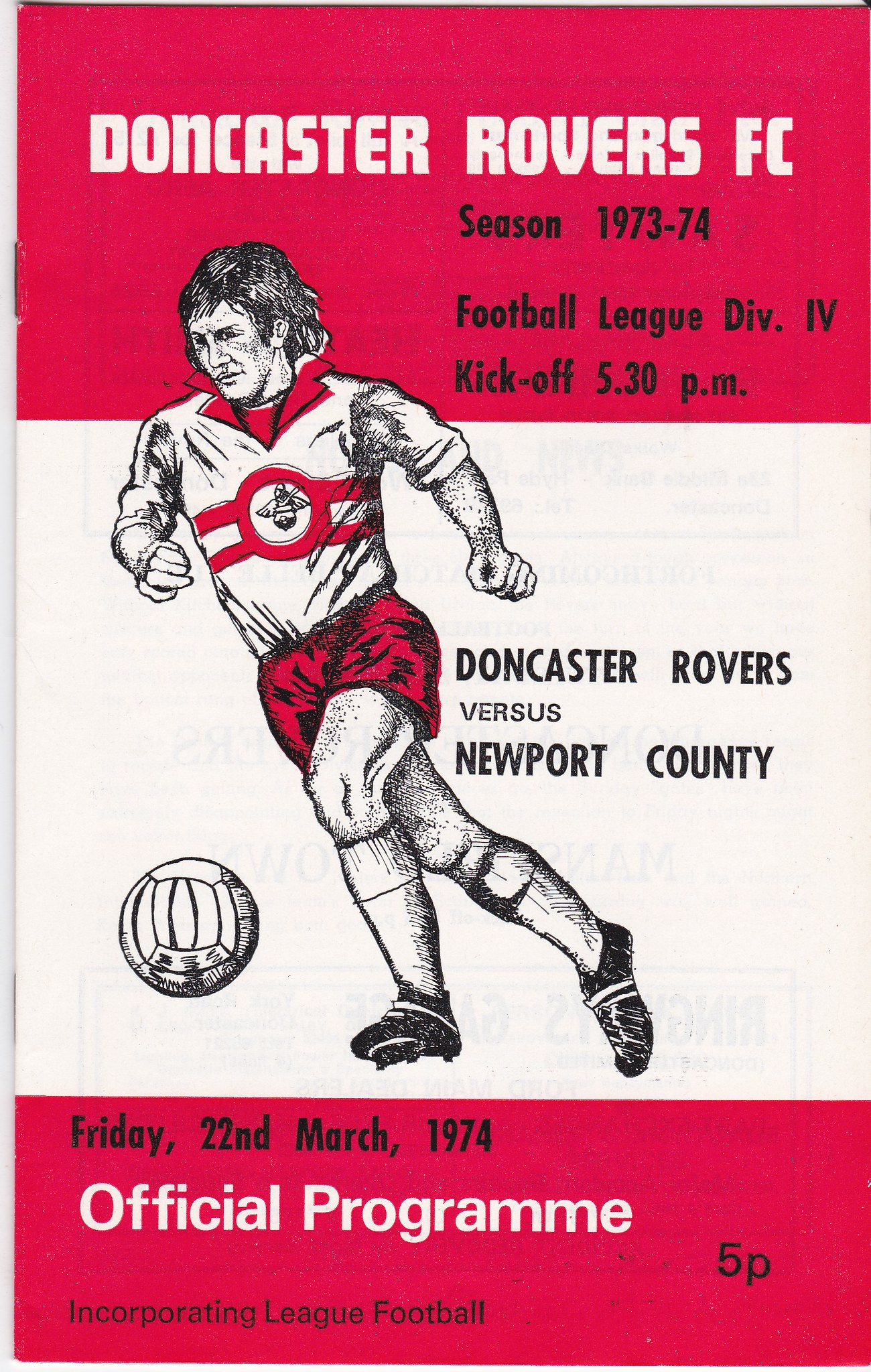The image is a detailed cover of a soccer program from the 1973-74 season of the Doncaster Rovers FC. The cover is primarily divided into three sections: a red stripe at the top, a white middle section, and another red stripe at the bottom. The top red stripe features white and black text that reads: "Doncaster Rovers FC," "Season 1973-74," "Football League Division IV," and "Kickoff 5.30 p.m." 

The middle section, set against a white background, prominently displays a colored pencil-style illustration of a soccer player in action, seemingly about to kick a soccer ball positioned below his right knee. The soccer player is depicted wearing a white t-shirt with a red collar and a red outlined circle over two red bars on the chest, paired with red shorts, socks, and athletic shoes. The text in this section states: "Doncaster Rovers" on the first line, "Versus" in smaller font on the second line, and "Newport County" on the third line.

The bottom red stripe lists in black text: "Friday, 22nd March, 1974," followed by "Official Programme" in bold white letters, and "Incorporating League Football" in smaller black text on the left. On the right side of this stripe, the price is shown as "5P."

Notably, the program cover also features two staples on the left, indicating it is a booklet for a sporting event.